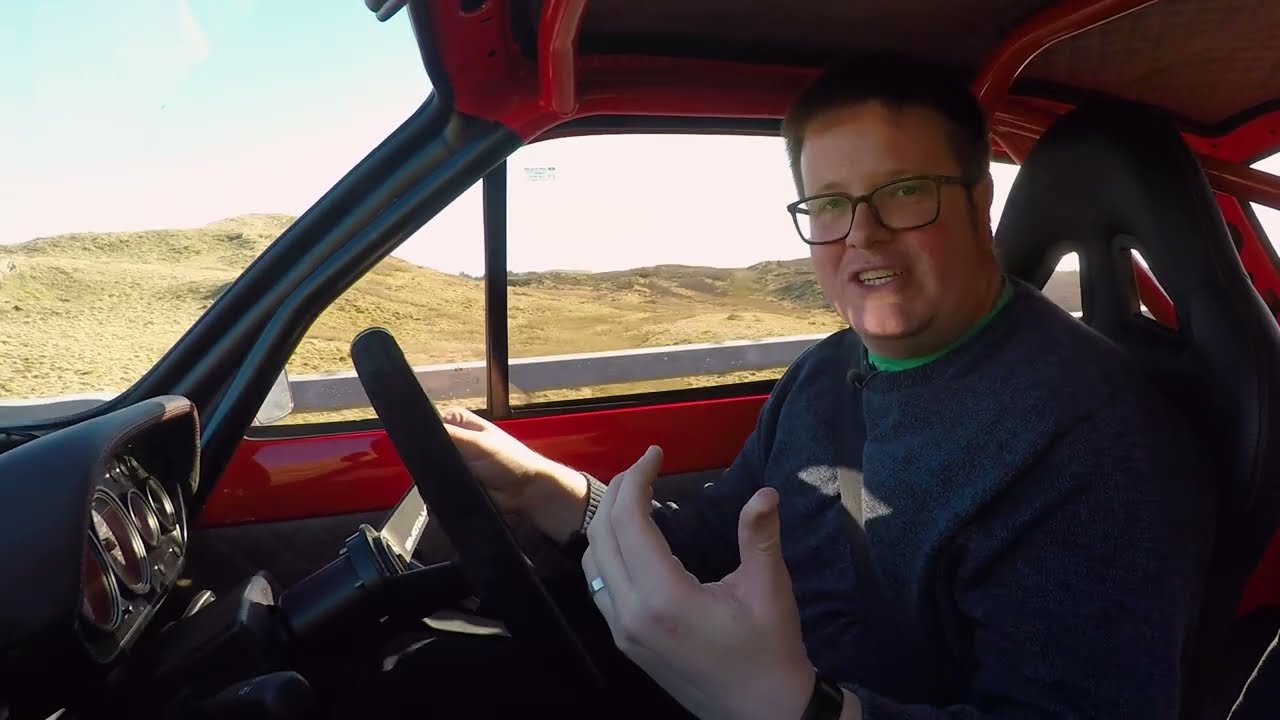The image features a middle-aged, slightly overweight man with glasses, wearing a blue sweater, driving a right-hand drive car, indicating he may be in the UK or a similar region. He is actively engaging in a conversation with the camera, holding the steering wheel with his right hand while gesturing with his left. The car’s interior is predominantly black with sporty features, including racing seats, a roll cage, a sporty steering wheel, and various gauges. Some red trim, possibly the roof and parts of the interior, contrasts with the black. Through the windows, the background reveals a desert-like landscape with yellow-brown dirt and sand, under a hazy blue sky. Additionally, a white handrail is visible alongside rolling hills made of either dry grass or dirt.